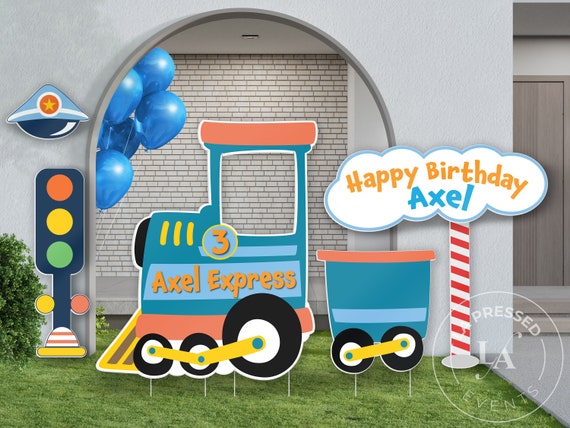In the image, we are outside in front of a house, visible by the gray stone wall with a gray archway and door on the right-hand side. The scene is set for a children's birthday party, suggested by the festive decorations occupying the tuft of grass. At the center of the lawn is a blue and orange cardboard cutout resembling a toy train, labeled "Axel Express 3," indicating possibly a third birthday. The train features additional vibrant yellow stripes and a circular blue backdrop behind the number three. 

To the train's right stands a barber-pole-like structure with red and white stripes supporting a large cloud-shaped sign bordered in blue. This sign reads, "Happy Birthday Axel" in orange and blue letters. Adjacent to these decorations, on the left, is a toy stoplight planted in the grass, showcasing red, yellow, and green lights. Blue balloons are also tied in this area, enhancing the celebratory atmosphere.

The backdrop includes a small shrub on the left near the gray brick wall, which helps frame the scene against the gray façade. Topping off the decor is a pirate hat placed over a lamp with a star design. The event's setup was orchestrated by Pressed LA Events, as indicated by their logo in a light round circular font.